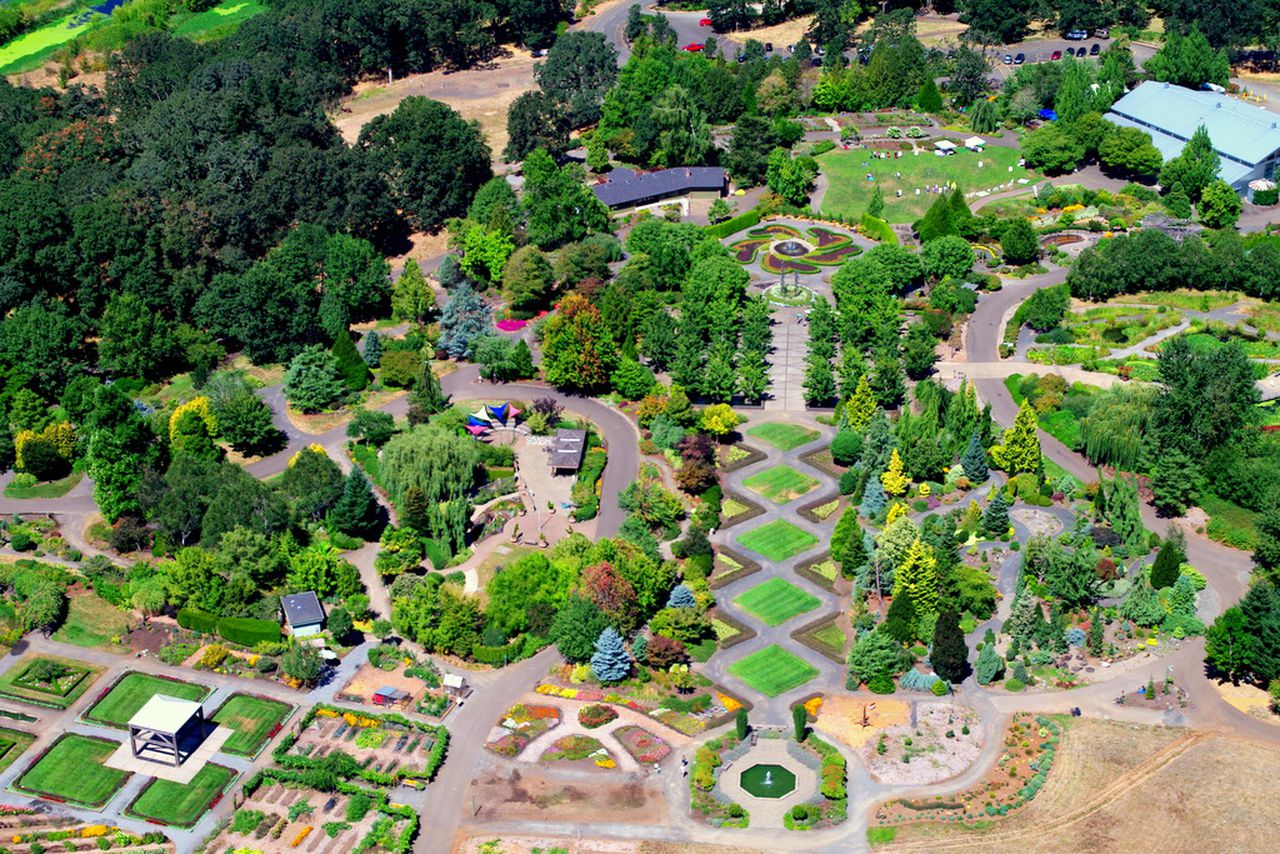The image depicts an overhead view of a meticulously landscaped garden area, characterized by a maze-like arrangement of both high and lower-growing trees. The trees, in shades ranging from dark to light green, serve as a lush backdrop to the scene. Prominent amongst the greenery are distinct patches of manicured lawns, interspersed with creatively shaped flowerbeds displaying vibrant red, yellow, green, and orange flowers.

Several buildings with flat rooftops can be seen nestled among the trees, including one with a blue roof, positioned toward the right of the frame. On the left-hand side, an auditorium-like building with a darker blue roof is also visible. An athletic field lies to the left of this building, where people can be seen gathered around small vendor tents scattered around the field's edge. 

In the upper right corner, there is a neatly organized parking lot filled with cars, while the lower left corner showcases four distinct patches of green grass surrounding a white-topped metal stage, approximately eight to ten feet off the ground.

Dominating the top middle section of the image is a circular roundabout containing additional green and brown grass patches. Decorative walking paths and possibly narrow roads crisscross the area, enhancing its park-like ambiance. Towards the lower center, rectangular hedges frame sections filled with diverse colored flowers, and a noticeable dirt patch bordered by hedges sits in the right corner of the image. An overarching sense of green prevails throughout, punctuated by the occasional yellowing tree, encapsulating the essence of a beautifully maintained garden park.